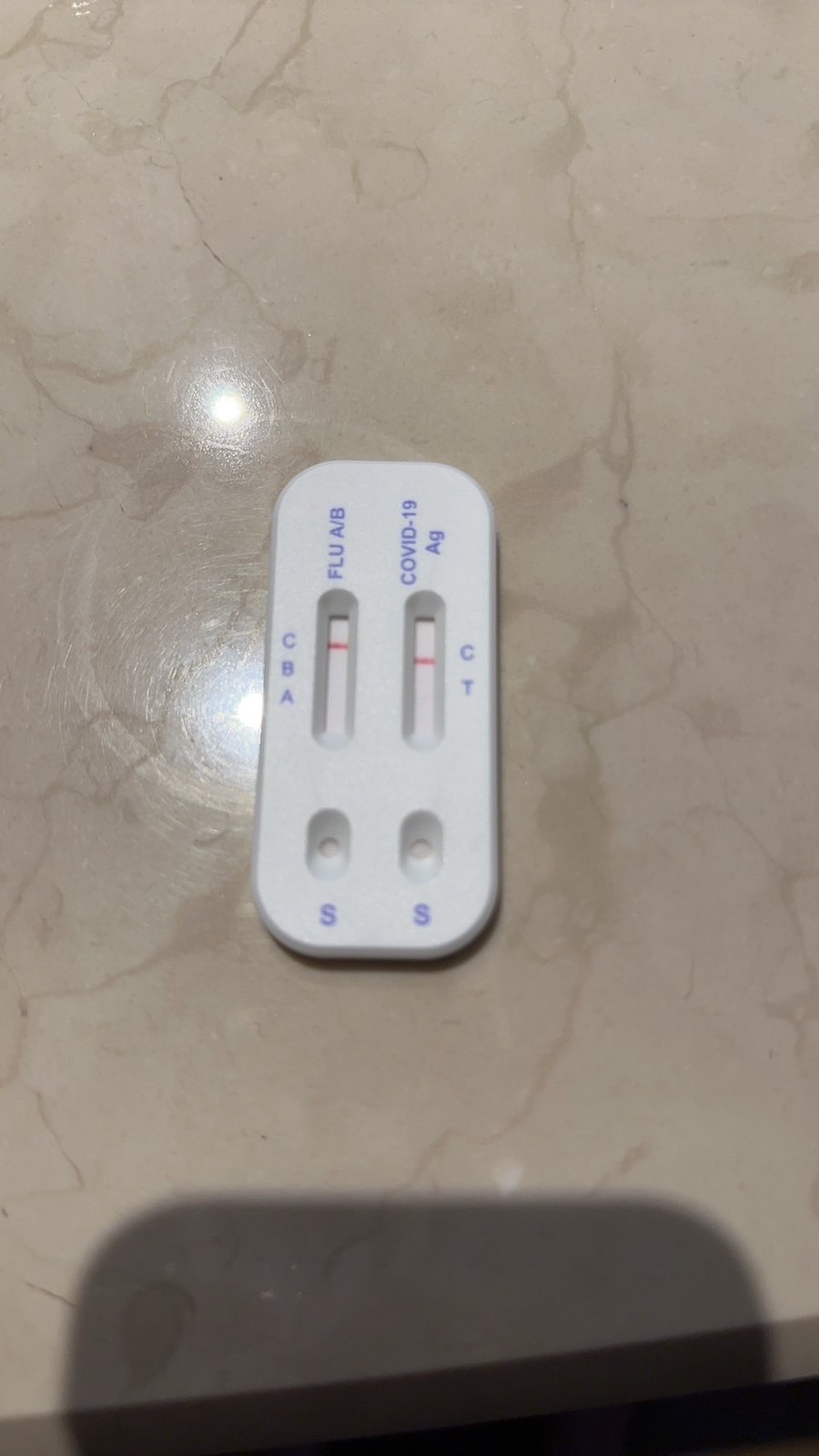The photo captures the top of a finely polished granite countertop, predominantly light beige with a scatter of darker beige accents. The surface gleams under illumination, with two distinct light reflections appearing as dots on the top left side of the image, approximately six inches apart. Centrally positioned on the countertop is a white, rectangular object, identified as a COVID-19 test. The test device is marked with "COVID-19" in bold letters, along with various labels. On one side, labeled "CBA," there is an oval-shaped indentation marked with a red line. The opposite side, marked "CT," also features a red line. Additionally, at the bottom are two smaller oval shapes labeled "SS," with all text rendered in blue. Below the test kit, only partially visible and blurred, is the edge of a dark, phone-like object.